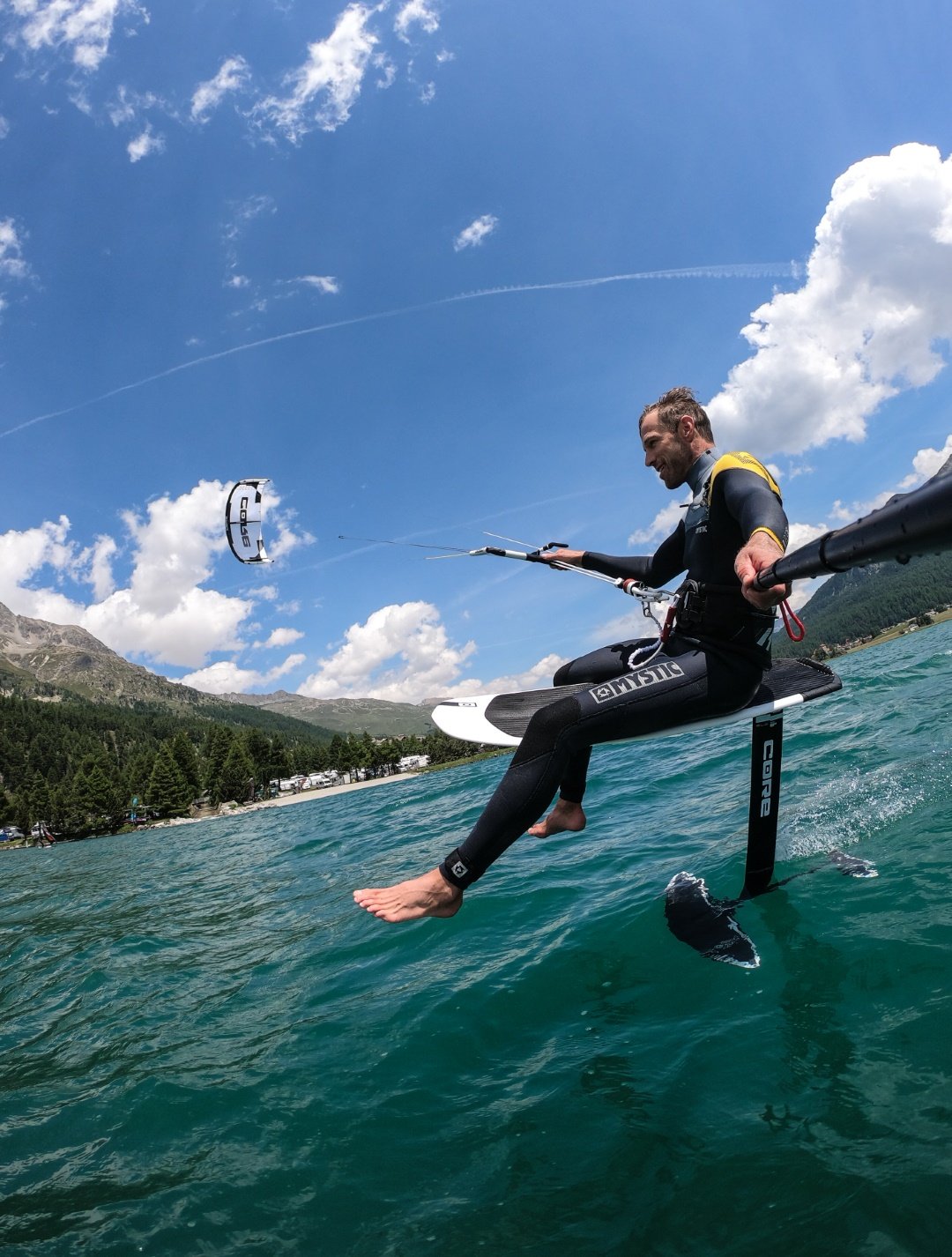This vibrant image captures a thrilling action moment of a man engaged in a water sport resembling wind gliding or parasailing. The scene shows him seated on an advanced two-level watercraft, with the top level appearing like a boogie board and the lower level connected by a vertical bar, reminiscent of a hammerhead-shaped surfboard beneath the water. He is holding a black bar in his right hand, which is connected to a fully extended parachute with black and white colors, visible towards the upper left of the image. In his left hand, he has a selfie stick, suggesting the photo could be taken with a GoPro.

The man sports a black wetsuit, with "Mystic" printed on the left outer leg, and has yellow accents on the shoulders. He is barefooted and bareheaded, with dark brown hair moving in the wind. Surrounding the action are serene green mountains and possibly a lake or a river—though it lacks the white-capping of ocean waves, the water has noticeable ripples.

In the expansive background, the sky is a deep, clear blue and filled with large, fluffy white clouds. There's also a contrail arching gracefully from left to right, partially obscured by clouds. The shoreline features buildings and homes, enhancing the picturesque setting of this adrenaline-fueled adventure.